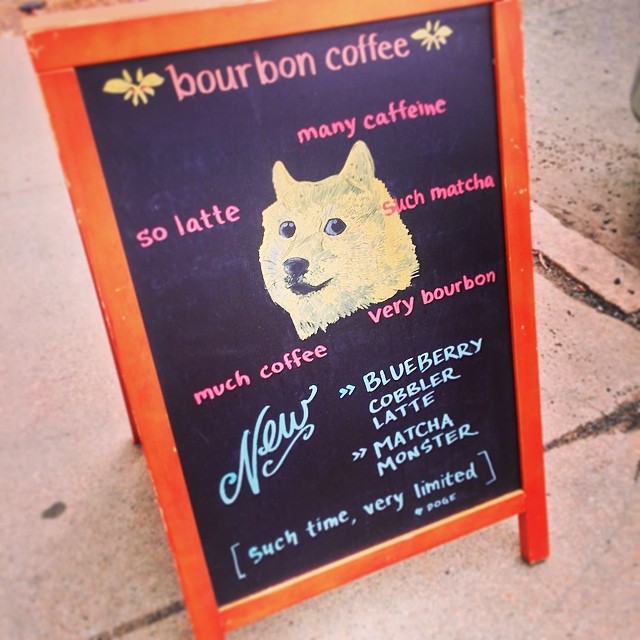The image is a photograph taken outside, showing a sidewalk chalkboard with a red easel frame. At the top of the chalkboard, written in pink lowercase letters, it says "bourbon coffee," flanked by small yellow butterflies. Central to the design is a stylized drawing of a Shiba Inu dog's head with dark eyes and a brown nose, surrounded by various phrases in pink chalk: "mini caffeine" at the top, "so latte" in the upper left corner, "such matcha" on the right, "much coffee" on the bottom left, and "very bourbon" in the bottom right. Below the dog's head is the word "new" in blue cursive followed by the names of limited-time drinks: "Cobbler Latte" and "Matcha Monster." The chalkboard is set up on the sidewalk, creating an inviting display for passersby.